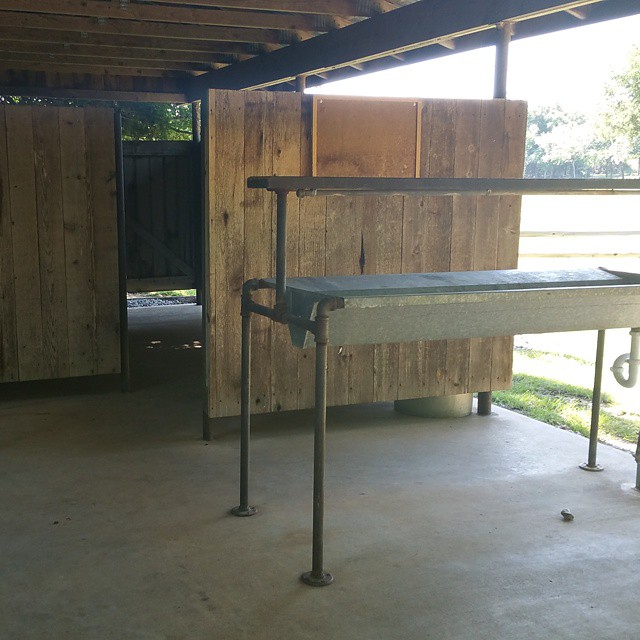The photograph showcases an open-air shed with a roof supported by unfinished wooden scaffolding and visible support beams, capturing an outdoor environment during the daytime. The upper right corner reveals a bright, sunny sky with scattered trees and patches of green grass beyond the structure. The shed's concrete flooring is partially enclosed by wooden walls, arranged to form an almost square shape with an opening at one corner, allowing a view of the outside. Dominating the foreground on the right side is a robust, installed metal desk or counter with four metal legs embedded into the concrete ground. The metal surface is partially covered by a piece of fabric or rubber, and a pipe extends down from the right side, suggesting it might be used as a tool table or workbench. The scene evokes a functional, semi-outdoor workspace blending natural and constructed elements.